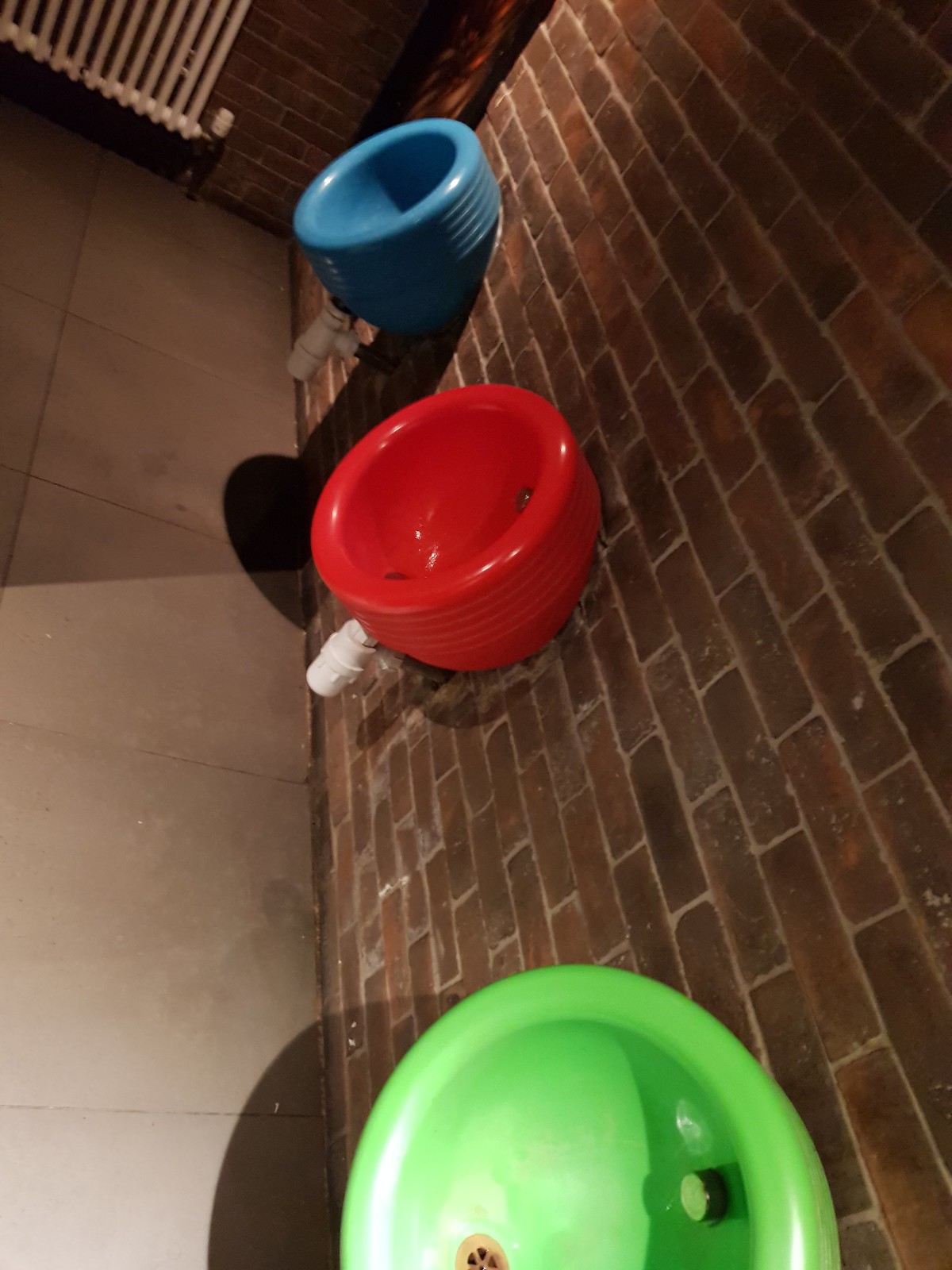The photograph, likely taken from a cell phone, depicts a slightly tilted scene of a public bathroom with a warm, reddish-brown brick wall to the right and a tiled, beige wall to the left. The floor, appearing to be gray or dark brown tile, is visible due to the image being rotated about 90 degrees. On the brick wall, three uniquely colored and circular urinals are mounted vertically. The urinal furthest back is blue, the middle one is red, and the nearest one is lime green. Each one has a white pipe protruding from its bottom, leading back into the wall. The urinals appear somewhat like cups with drains at their bases and silver flush buttons on their sides. Positioned higher up in the top left of the image is an old-fashioned white radiator, contributing to the old-school aesthetic of the room. The entire scene is lit from above, casting shadows and highlighting the contrast between the brick and tiled surfaces.